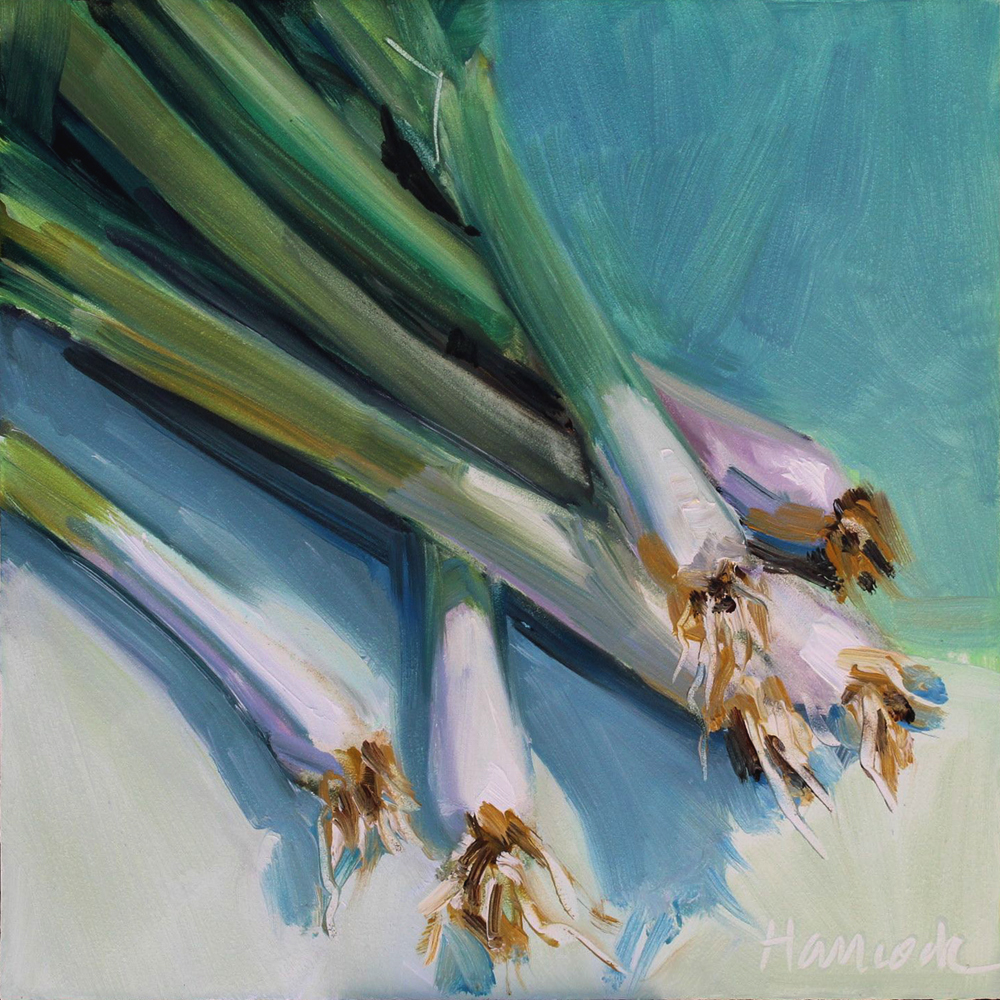This is an oil painting of green onions, or scallions, with the artist's signature "HANIOK" in the bottom right-hand corner. The composition features the white-bottomed scallions prominently, with their brownish-tan roots clearly visible, snapped off at the ends. The green stalks of the onions fan out and overlap naturally, displaying various natural shades of green and blending seamlessly into the white bases. The background reveals visible brush strokes and a blend of blues and greens at the top, suggesting a wall, while the middle to the lower section transitions into a white and slight grayish shadow to mimic the surface where the scallions lie. The delicate blending of colors and the skilled rendering of shadows add a realistic depth to the scene, making the vegetables appear almost lifelike.